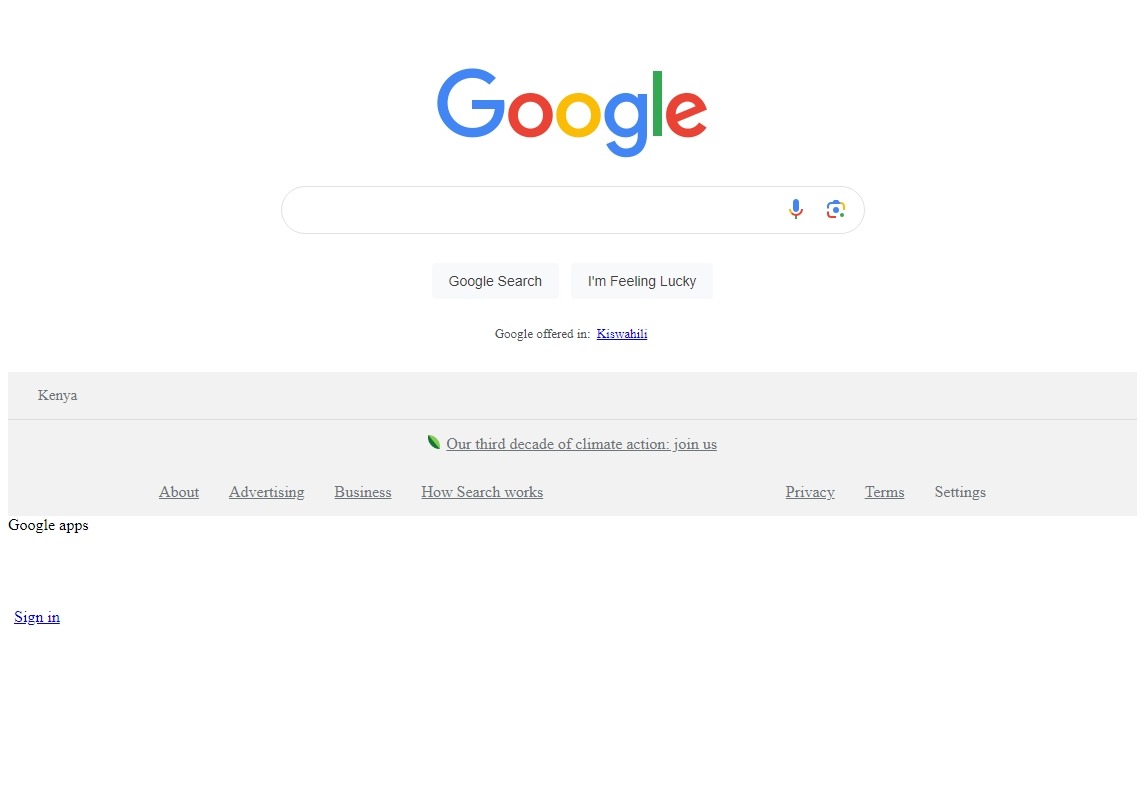The image features a minimalist design set against a clean, white background. At the top, prominently displayed, is the iconic Google logo, composed of its characteristic colorful letters— a blue uppercase "G", followed by a red upper-case "O", a yellow upper-case "O", a blue lowercase "g", a green lower-case "l", and finally, a red lower-case "e". 

Beneath the Google logo lies the familiar search bar, representing the core functionality of the search engine. This search bar is flanked by a microphone icon on the left, indicative of voice search capabilities, and an image icon on the right, suggesting an option for image-based searches. Directly below the search bar, two buttons are visible— the first, labeled "Google Search," and the second, labeled "I'm Feeling Lucky."

Underneath these primary elements, small text reads, "Google offered in" followed by what appears to be a blue hyperlink word that starts with the letter "K", though its exact nature is unclear due to the blurriness. Additionally, a light gray rectangular box reveals "Kenya," which is further underscored by a light gray horizontal line stretching across the page. An adjacent message promotes environmental awareness with the text "Our third decade of climate action, join us."

At the very bottom of the image, there is a series of navigational links in light gray text: "About," "Advertisement," "Business," "How Search Works," "Privacy," "Terms," and "Settings," offering users quick access to various informational and account-related resources.